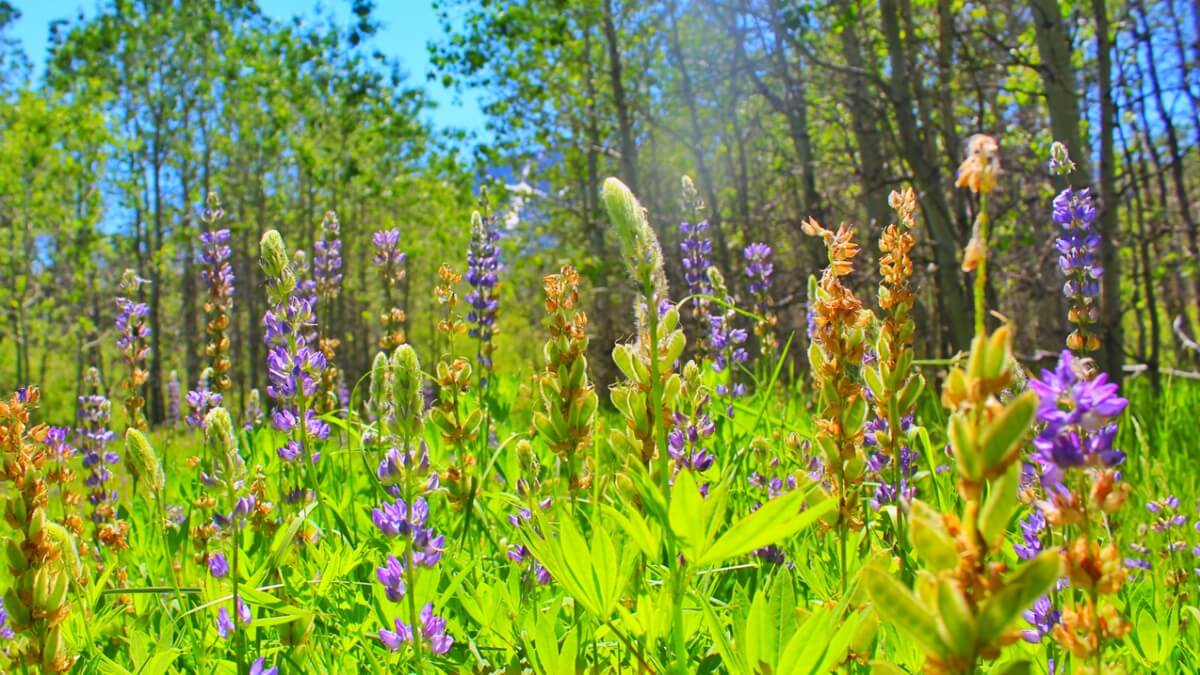This vibrant, professional photograph captures a close-up of a colorful flower field on a bright, sunny spring day. Dominated by purplish lavender blooms, the image also showcases pops of yellow and orange buds against a sea of vibrant, chartreuse green leaves. The clear blue sky overhead contrasts beautifully with the forest of tall, slender trees, their green leaves glowing in the sunlight and trunks just visible in the background. The flowers in the foreground are sharply in focus, their vivid hues accentuated by the high contrast and saturation, while the background softly blurs, emphasizing the density of the foliage and giving a dreamy quality to the scene. There are no humans or animals present, allowing the natural beauty to stand out effortlessly.